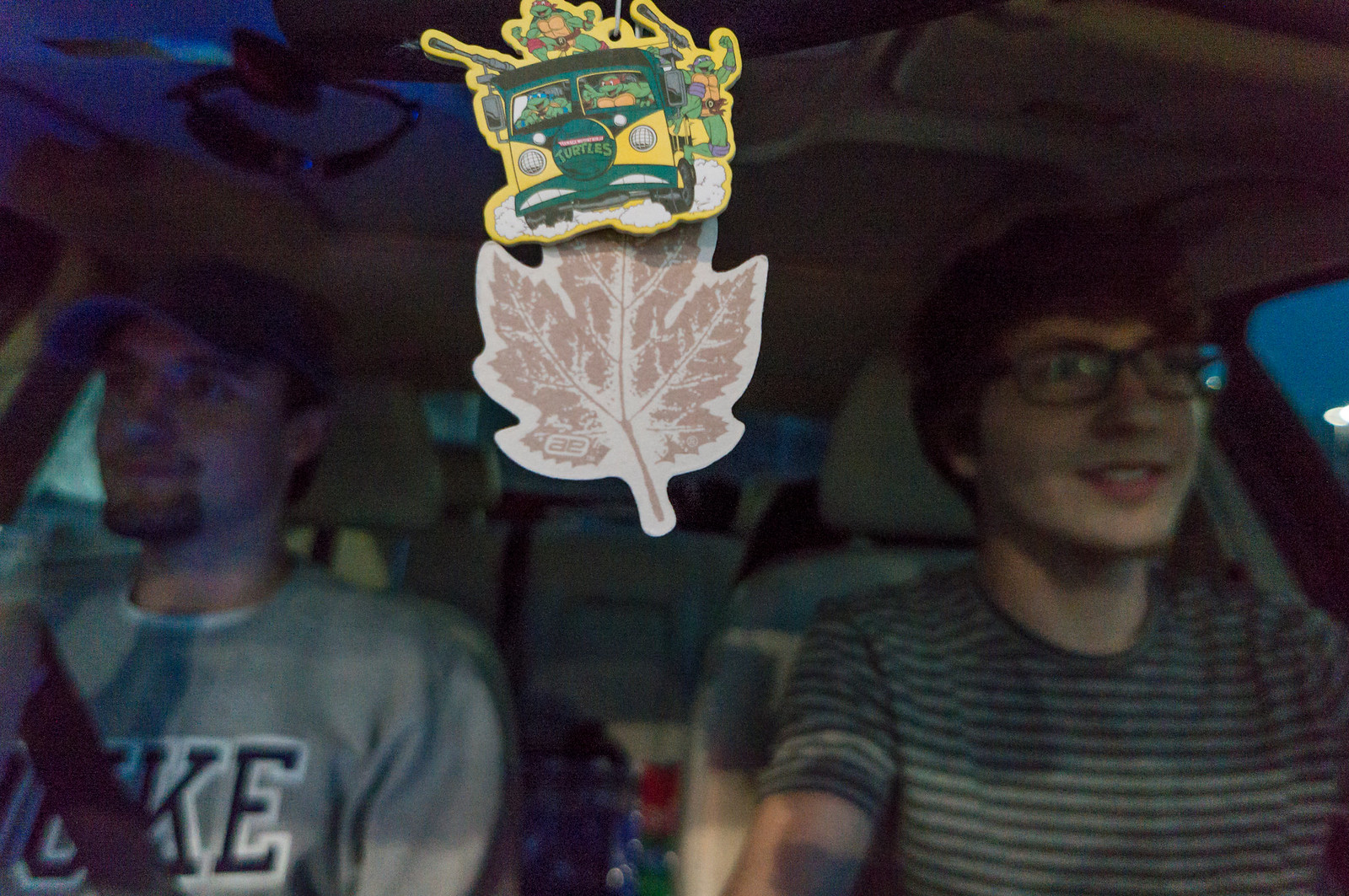This slightly blurred photograph captures an interior view from the dashboard of a car, primarily focusing on two men seated in the front. The foreground is dominated by two air fresheners hanging from the rearview mirror—the first is a Teenage Mutant Ninja Turtles-themed one, brightly colored in yellow and green, depicting the turtles in their van; the second is a brown maple leaf. The driver, a young Caucasian male with short brown hair and black-brimmed glasses, is wearing a green striped shirt and smiling, although he doesn't appear to be wearing a seatbelt. In the passenger seat sits another man, also Caucasian, dressed in a gray Duke sweatshirt with blue lettering outlined in white, a white shirt underneath, and a blue baseball cap. He has a goatee and is wearing a seatbelt. The image hints at some food items or drinks placed in the rear seats behind them.